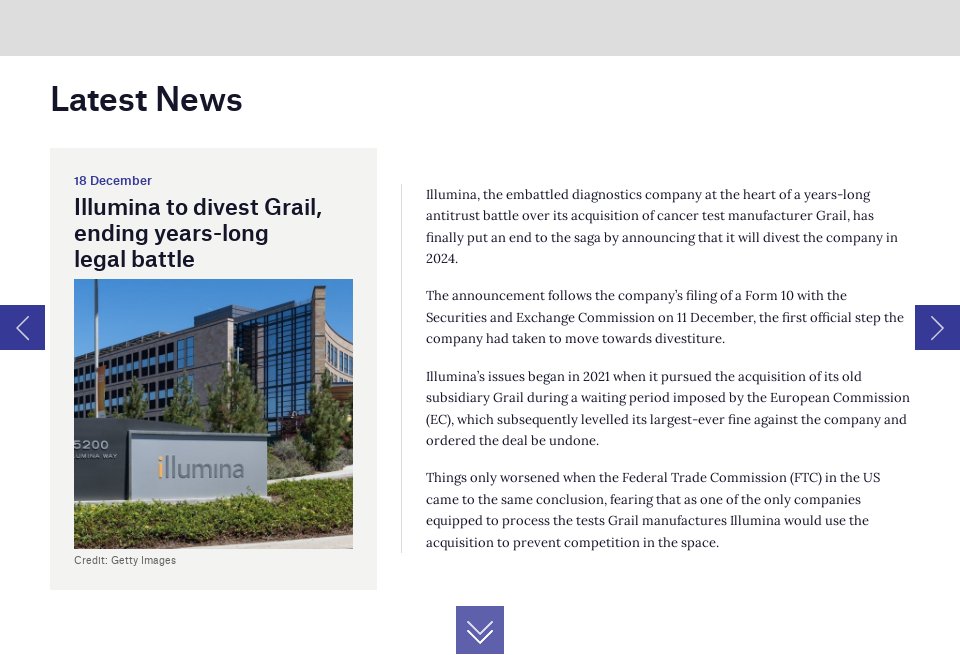**Caption:**

On the website "Latest News," prominently displayed in bold at the top left, there is a detailed update dated December 18th regarding Illumina's decision to divest Braille, concluding a protracted legal dispute. The webpage features a clean design with a white background and black text, ensuring readability.

A photograph of Illumina's headquarters accompanies the article. To the right, there is an in-depth narrative detailing Illumina's embattled history. Illumina, a diagnostic company central to a prolonged antitrust conflict, has announced it will divest Braille in 2024. This follows their filing of Form 10 with the Curating Change Commission on December 11th, marking the first formal step towards divestiture.

Illumina's troubles began in 2021 when they attempted to acquire their subsidiary, Braille, during a waiting period mandated by the European Commission (EC). The EC subsequently imposed significant fines, demanding the acquisition to be reversed. The situation deteriorated when the US Federal Trade Commission (FTC) echoed the EC’s concerns, concluding that Illumina's acquisition of Braille hindered competition in the cancer test-manufacturing sector.

Navigation on the page is facilitated by purple forward and back buttons on either side and a double arrow button at the bottom for scrolling down.